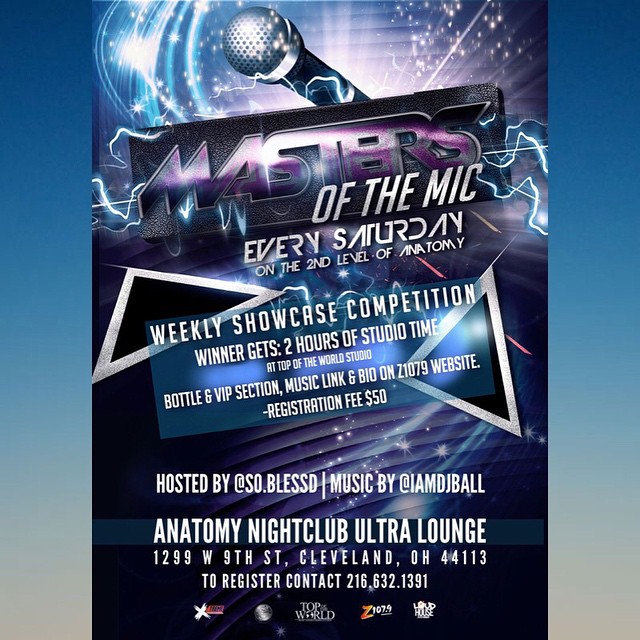Set against a blue background, this detailed and vibrant poster promotes a weekly singing competition called "Masters of the Mic," held every Saturday on the second level of Anatomy Nightclub Ultra Lounge, located at 1299 West 9th Street, Cleveland, Ohio 44113. The top of the poster features a large microphone surrounded by silver swirls, stars, and electric bolts, creating a dynamic and eye-catching visual. The title "Masters of the Mic" is displayed prominently beneath the microphone, with the phrase "every Saturday on the second level of Anatomy" clearly stated below it.

The center of the poster announces the "Weekly Showcase Competition" in white letters, offering enticing rewards for the winner: two hours of studio time at Top of the World Studio, a bottle and VIP section, and a music link and bio on the Z 107.9 website. The registration fee for participants is $50. The event is hosted by @so_blessed with music by @IAmDJBall. At the very bottom, the poster reiterates the location and contact information for registration, providing a contact number: 216-632-1391. Additionally, logos of sponsors such as Z 107.9 and Top of the World, among others, are displayed, though some are less identifiable. This detailed flyer creates a clear and compelling invitation to aspiring artists and music enthusiasts.